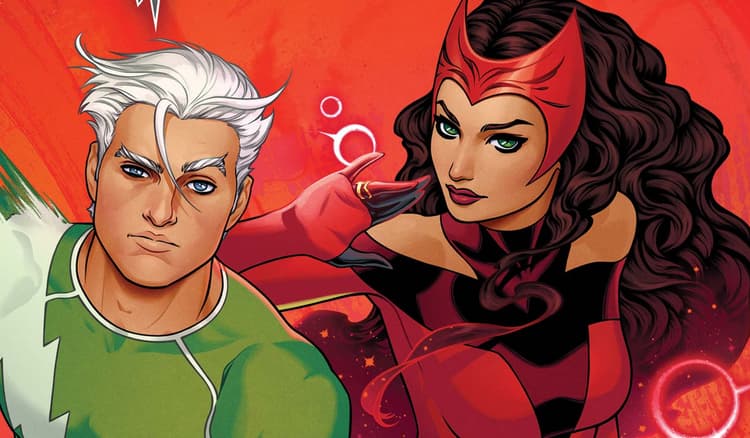This image is a digital illustration, reminiscent of a cartoon TV show or a comic book, with a rectangular layout that is wider than it is tall. The background is a vibrant red, creating a striking backdrop for the two main characters depicted in the scene. On the left side stands a man with a medium skin tone, donning a green and white suit that features a lightning design cascading from his right shoulder across his chest. His short, feathered white hair is complemented by a wispy bang across his forehead, and he has gray eyebrows and blue eyes. 

To the right of the man is a woman dressed in a striking red suit, which includes black and purple elements. She has long, wavy brown hair and green eyes. Her headgear resembles a mask with double ear-like shapes, perched atop her head. She wears distinctive red gloves that have pointed tips, some of which are black, and she sport a gold ring on her ring finger. In the bottom right corner of the image, there is a round logo, although the text within it is not legible. This carefully crafted illustration highlights the detailed and vibrant design of these two superhero-like characters.